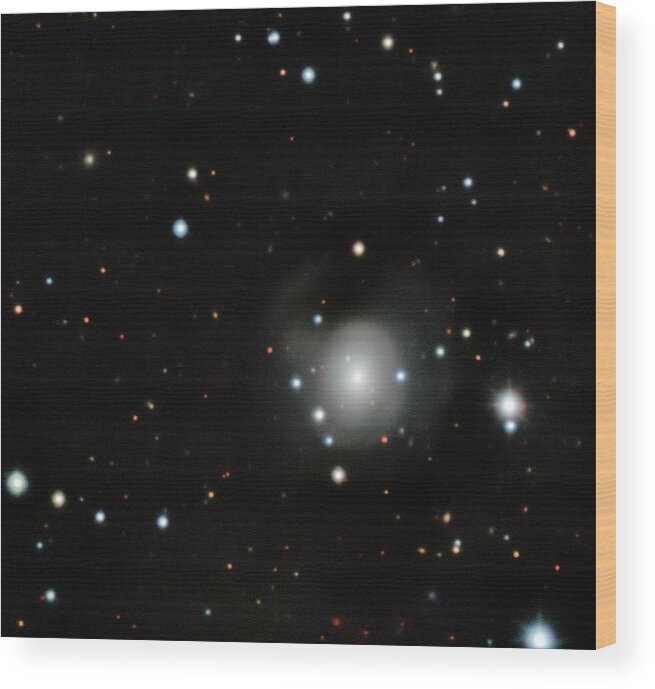The image features a black-painted wooden board with a smooth, consistent surface. Scattered across the dark backdrop are multi-colored, glowy dots resembling stars, in shades of blue, yellow, white, and pink. These stars vary in brightness and size, adding to the dynamic, celestial feel of the artwork. Dominating the center is a particularly bright, white cluster that radiates outward, creating a hazy, cloud-like effect reminiscent of the Milky Way. The right edge of the image reveals the wood grain and a light beige color of the underlying wood, adding a tactile, three-dimensional quality to the piece. This thoughtfully crafted artwork captures the beauty and mystery of the night sky, making for a striking visual experience.